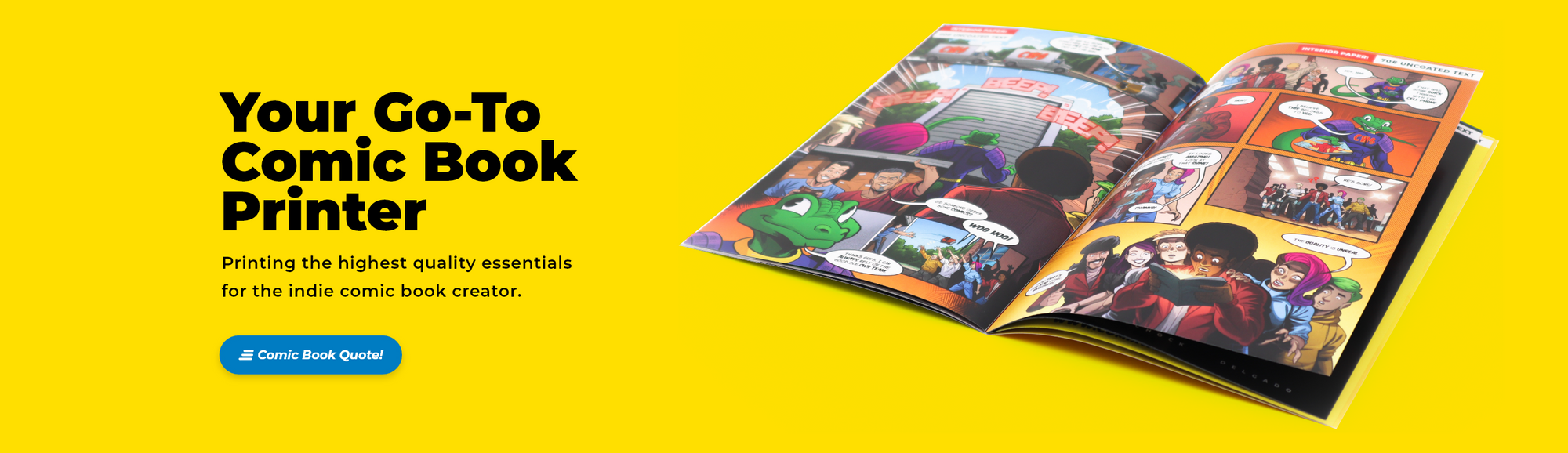The advertisement features a bright yellow background with black text on the left side that reads, "Your go-to comic book printer, printing the highest quality essentials for the indie comic book creator." Below the text, there is a prominent blue button labeled "comic book quote!". To the right, an open, colorful comic book lays flat, showcasing vivid illustrations that include a green snake or frog, a group of people, and a staircase. The comic book adds a dynamic splash of color, enhancing the overall eye-catching design of the advert. The ad is clearly targeted toward indie comic book creators looking for high-quality printing services.